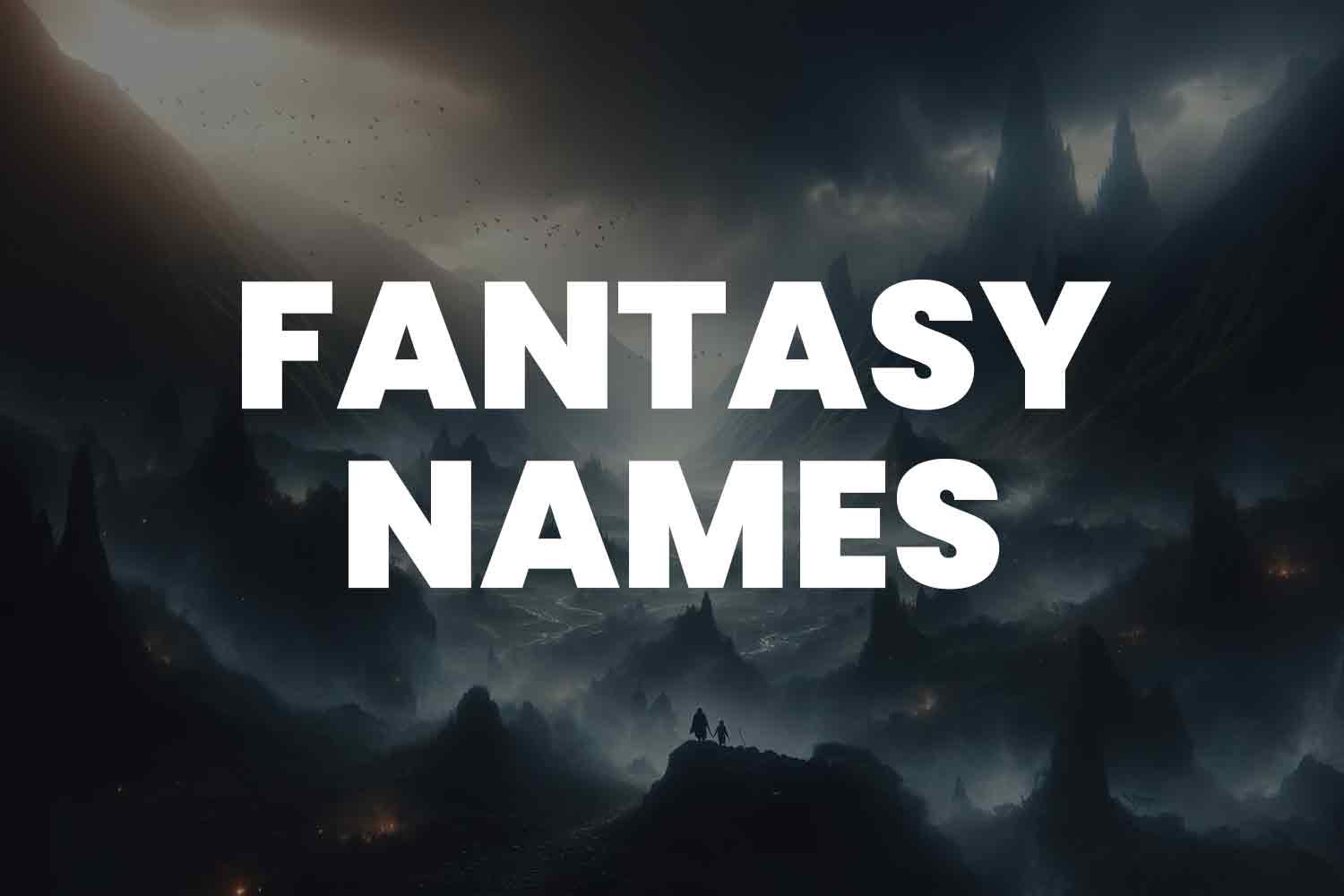This rectangular, wide vertical screenshot showcases a computer-generated, otherworldly fantasy landscape dominated by dark, craggy mountain peaks and an ominous, foggy atmosphere. The background is enveloped in dense fog, with hints of dark gray clouds and a slightly lighter sky illuminated subtly in the upper left corner. The scene is painted in largely black and dark gray hues, with some birds depicted flying across the sky. In the nearest foreground, two silhouetted human figures, one appearing taller and cloaked and the other shorter, stand on a rocky outcropping. Adding to the eerie ambiance, distant fires seem to flicker in the valley between the mountains. Boldly overlaid in white, large, sans-serif, all-caps text across the center of the image are the words "FANTASY NAMES," possibly indicating the header for a list of fantasy names on a website.